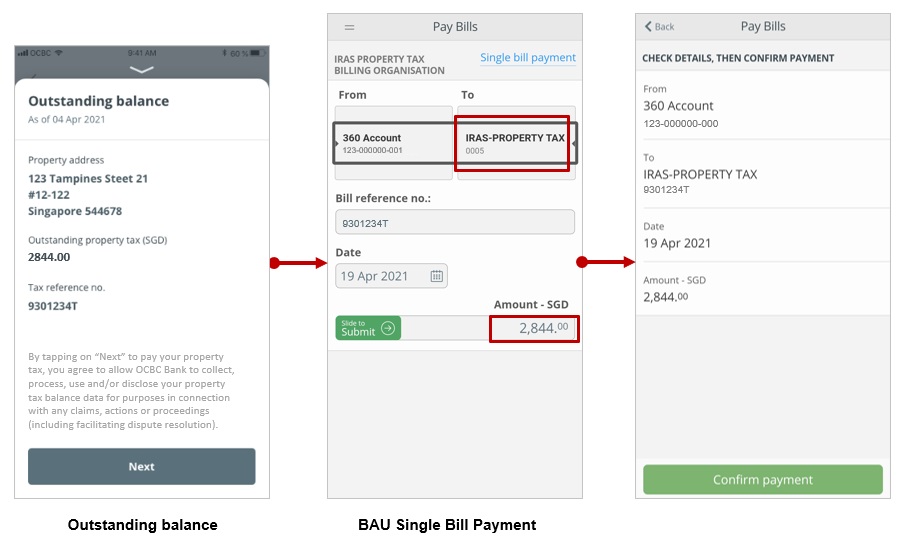The image features a compilation of three distinct smartphone screen captures presented in an editing software, where red boxes and lines have been added to direct attention to important elements.

1. **First Screenshot (Left):**
    - **Focus:** Outstanding balance of property tax.
    - **Highlighted Text:** "Outstanding property tax: $2844.00."
    - **Indicators:** A red box around the outstanding balance amount and a red arrow pointing towards the next screenshot.
    - **Addition:** At the bottom of this screenshot, it is labeled "Outstanding balance."

2. **Second Screenshot (Middle):**
    - **Focus:** Pay bills section for 360 account.
    - **Highlighted Texts:**
        - "IRAS-PropertyTax000015" highlighted by a red box.
        - The amount "$2844.00" also highlighted with a red box.
    - **Indicators:** A green "Submit" button is noted to the left of the amount. A second red arrow points towards the third screenshot.

3. **Third Screenshot (Right):**
    - **Focus:** Payment confirmation details.
    - **Highlighted Elements:**
        - Payee: "IRS-PropertyTax."
        - Date: "19th April 2021."
        - Amount: "$2844.00."
    - **Indicators:** Details include the payment source "360 account 123.0000.000." At the bottom of this screenshot resides a green "Confirm Payment" button.

This detailed composite walkthrough clearly guides the user through the process of paying an outstanding property tax bill, from viewing the balance to confirming the payment.